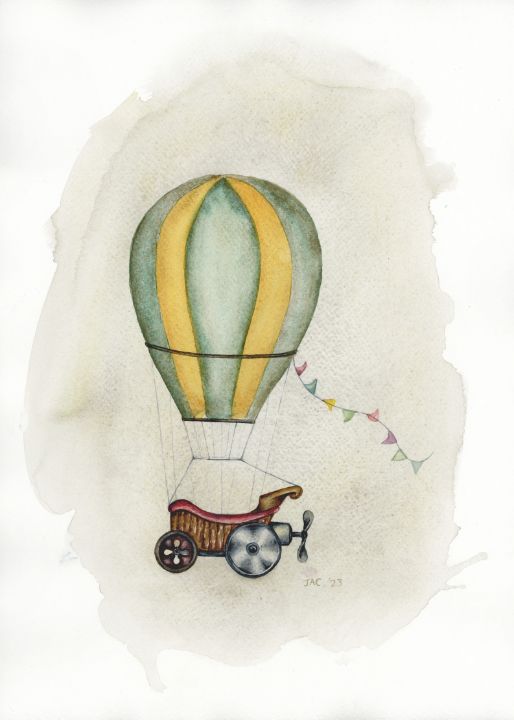The image is a detailed watercolor painting of a whimsical hot air balloon with green and yellow stripes. The balloon is tethered to a wagon-like carriage that resembles a chariot, featuring a small button-shaped front wheel and a larger solid metal rear wheel, both silver and black. The carriage is rendered in brown with red trim, and a basic fan blade propeller is mounted at the back, suggesting the ability to steer. A string of colorful triangular flags in pink, blue, yellow, and green trails from the balloon. The painting includes the artist's initials, JAC, and the year 2023, indicating it was either created or finished in that year. The artwork is set against a simple white background, enhancing the vibrant colors and delicate brush strokes.